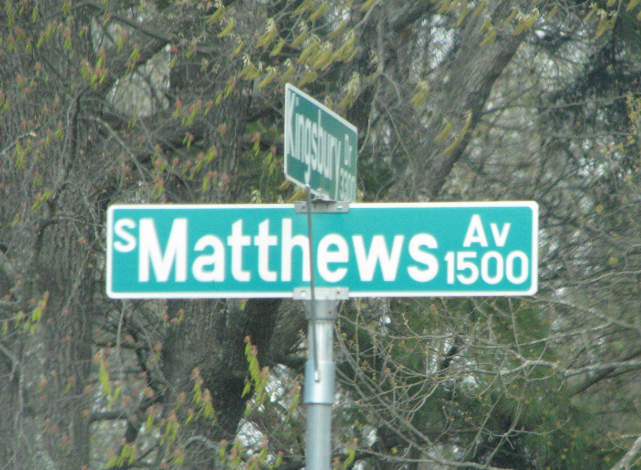This image features a street sign mounted on a silver metal pole. The prominent horizontal sign reads "South Matthews Avenue" and indicates the 1500 block. The intersecting street sign is partially obscured and angled away from the camera, making it difficult to decipher completely, though it appears to read "Keensbury Drive" with a designation of 3300. The background includes a large, mature tree with numerous branches, many of which seem barren and lifeless, giving the scene a somewhat bleak appearance. The overcast sky, visible through the sparse tree branches, enhances the overall somber mood of the photograph.